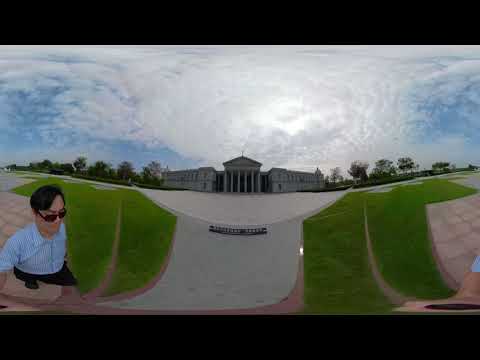In this wide-lens, daylight panoramic photo, a man, who appears to be of Asian descent, is captured walking in the bottom left corner. He is wearing sunglasses, a light blue button-up shirt, and black slacks. The setting is outdoors along a grass path leading to a central government building or courthouse that features Roman-inspired architecture, complete with columns and a triangular pediment. The expansive front courtyard is paved with light gray pavers, surrounded by a grassy area. The sky above is mostly covered with clouds, although the sun is attempting to peek through, creating a dramatic, overcast atmosphere. The photo's borders are solid black, framing this elegant scene with a palette of colors including black, blue, white, gray, green, maroon, tan, orange, and red.